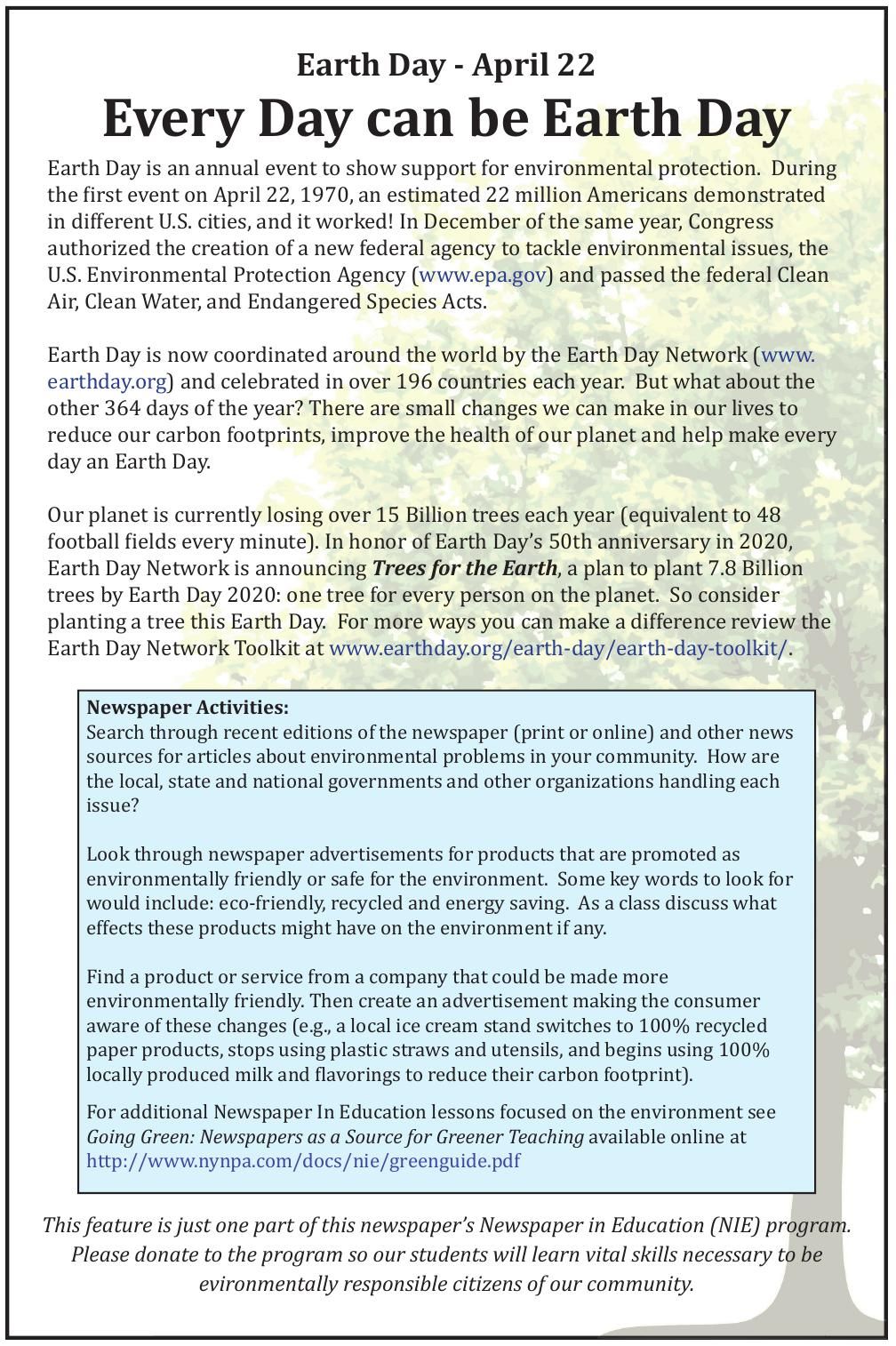**Earth Day**

**April 22nd: Every Day Can Be Earth Day**

**Earth Day is an annual event to show support for environmental protection. During the first event on April 22nd, 1970, an estimated 22 million Americans demonstrated in different US cities. In December of the same year, Congress authorized the creation of a new federal agency to tackle environmental issues, the US Environmental Protection Agency (www.epa.gov), and passed the Federal Clean Air, Clean Water, and Endangered Species Act. Earth Day is now coordinated around the world by Earth Day Network (www.earthday.org) and celebrated in over 196 countries each year. But what about the other 364 days of the year?**

**There are small changes we can make in our lives to reduce our carbon footprints, improve the health of our planet, and help make every day Earth Day. Our planet is currently losing over 15 billion trees each year, equivalent to 48 football fields every minute. On Earth Day's 50th anniversary in 2020, Earth Day Network announced "Trees for the Earth," a plan to plant 7.8 billion trees.**

**In collaboration with our Newspaper In Education (NIE) program, we are dedicated to providing students with the knowledge and skills crucial for becoming environmentally responsible citizens. Your donations to the program can help shape the future of our community.**

### Newspaper Activities

[Access more resources and activities](#)

---

**This feature is just one part of our Newspaper in Education (NIE) program. Please donate to support the program so our students can learn the vital skills necessary to be environmentally responsible citizens of our community.**

![Image of a tree with green leaves.]